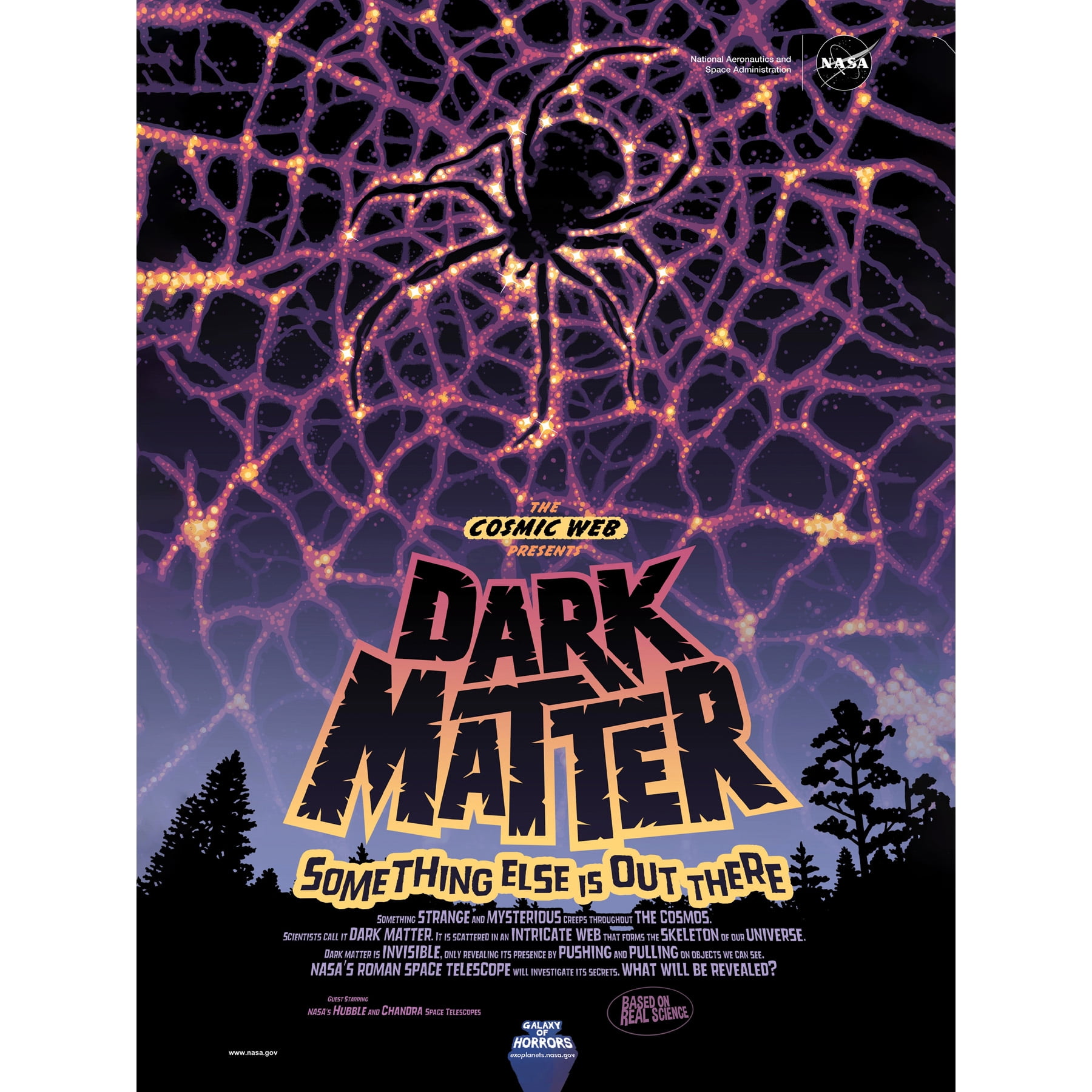The movie poster depicts a captivating night sky, shaded in deep purples and blues, adorned with an intricate spider web made of glowing stars connected by strands in purple and pink hues. In the middle of this cosmic web crawls a massive black spider, symbolizing the mysterious essence of dark matter. Crowning the upper section of the poster, the NASA logo and the text "National Aeronautics and Space Administration" embellish the top right corner, underlining the scientific intrigue of the theme. Dominating the poster's center, bold black text with an orange and yellow gradient outline proclaims, "The Cosmic Web Presents Dark Matter." Beneath, in contrasting black text with a gold outline, the ominous phrase "Something Else is Out There" hovers. Further down, nestled among the silhouettes of dark trees against the night, small text reads, "Something strange and mysterious creeps throughout the cosmos. Scientists call it Dark Matter. It is scattered in an intricate web that forms the skeleton of our universe. Dark Matter is invisible, only revealing its presence by pushing and pulling on objects we can see. NASA's Roman Space Telescope will investigate its secrets. What will be revealed?" The combination of stellar visuals and intriguing text promises an exploration into the enigmatic and unseen forces shaping our universe.